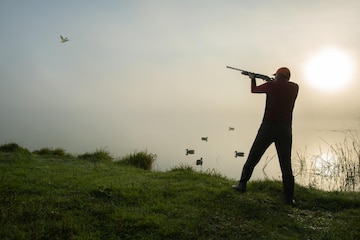In this atmospheric outdoor photograph, a man stands prominently on a grassy hill, positioned on the right side of the image. He's holding a rifle, aiming upward toward the upper left-hand corner of the frame where a white bird flies. Dressed in red clothing and a baseball cap, his silhouette is slightly obscured by the approaching evening light. The sky is overcast and carries a foggy ambiance, while the vibrant white-yellow sun peeks through the clouds from the upper right. Behind the man, a peaceful lake stretches out, dotted with a group of five ducks swimming leisurely. Overall, the scene blends the serene natural elements of the grassy hill and tranquil water with the tense moment of the man readying to shoot.